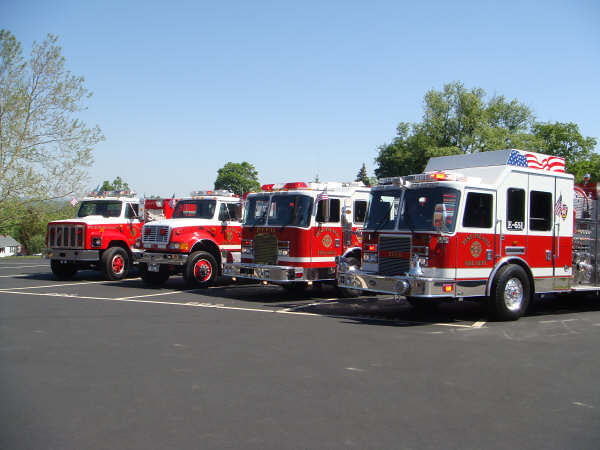In this photograph taken outdoors, four red and white fire trucks are parked in a parking lot, each occupying its own parking space though they appear slightly askew. All the trucks share a similar color scheme: the bottom half is red, the top half white, with a white stripe near the bottom and shiny silver bumpers. The first truck, labeled E65L, prominently features an American flag on its roof. The two closest fire trucks have flat noses while the two further away have bonnets. Overhead, the sky is clear and blue, and in the background, four trees of varying sizes are visible. On the left side of the image, a white house with a gray roof can be seen in the distance, accompanied by a sparse green tree in front, leaning to the right. Additionally, a larger, fuller tree on the right side and another smaller but equally dense tree further in the background complete the scene, indicating a sunny day with vibrant elements both near and far.